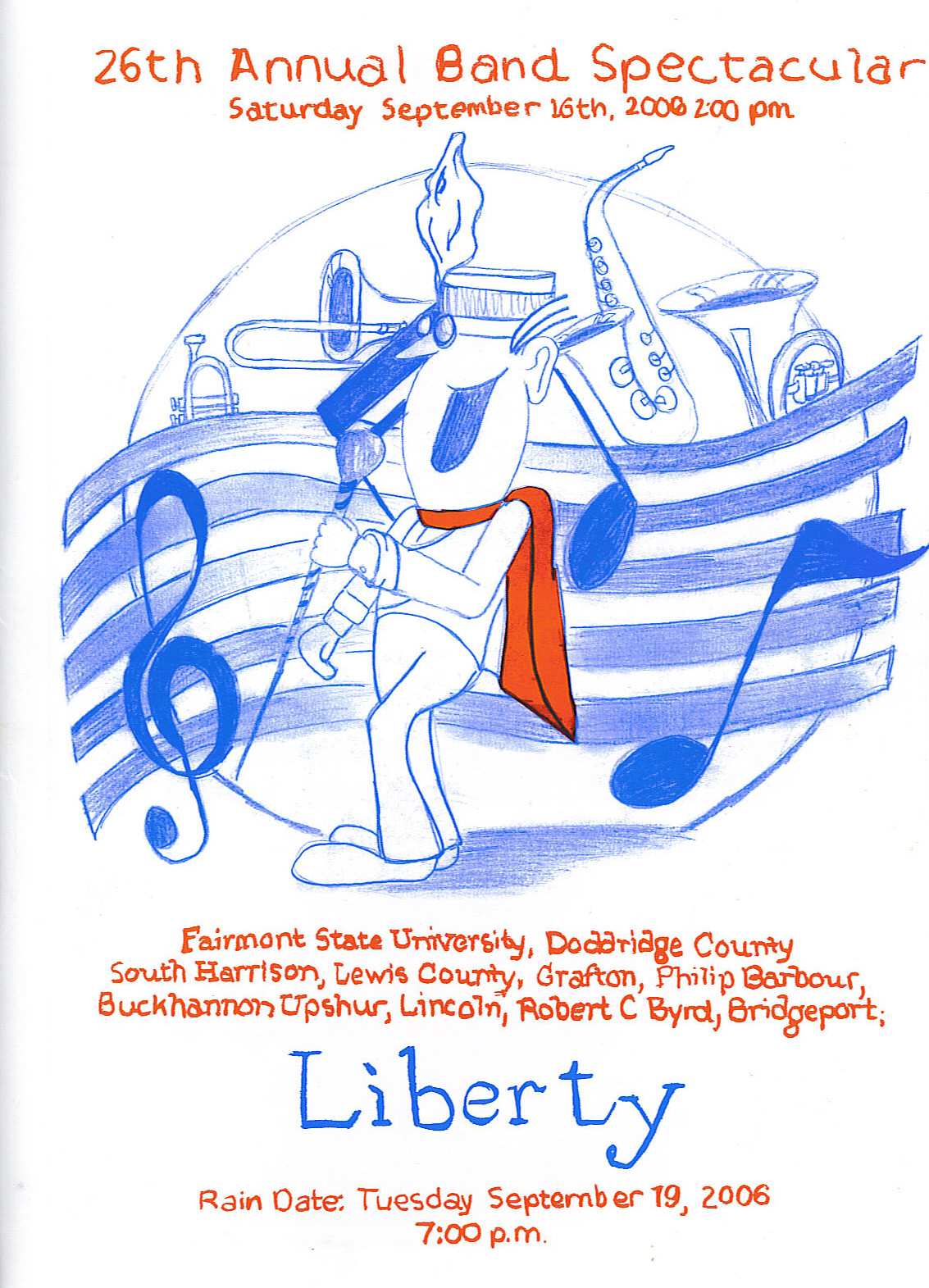This white poster advertises the 26th Annual Band Spectacular, happening on Saturday, September 16th, 2006, at 2 p.m. The event name and date are prominently featured at the top in red letters. At the center of the poster, there's a detailed illustration: a cartoony silhouette of a band leader wearing a red cape and holding a baton, with a backdrop of musical instruments including saxophones, tubas, and horns encased in a circle. Flowing stripes and music symbols add a lively touch to the design. Below this illustration, the participating groups are listed in red ink: Fairmont State University, Doddridge County, South Harrison, Lewis County, Grafton, Philip Barbour, Buchanan Upshur, Lincoln, Robert C Byrd, and Bridgeport, with the word "Liberty" in blue ink underneath. The rain date is also noted in red ink as Tuesday, September 19th, 2006, at 7 p.m.